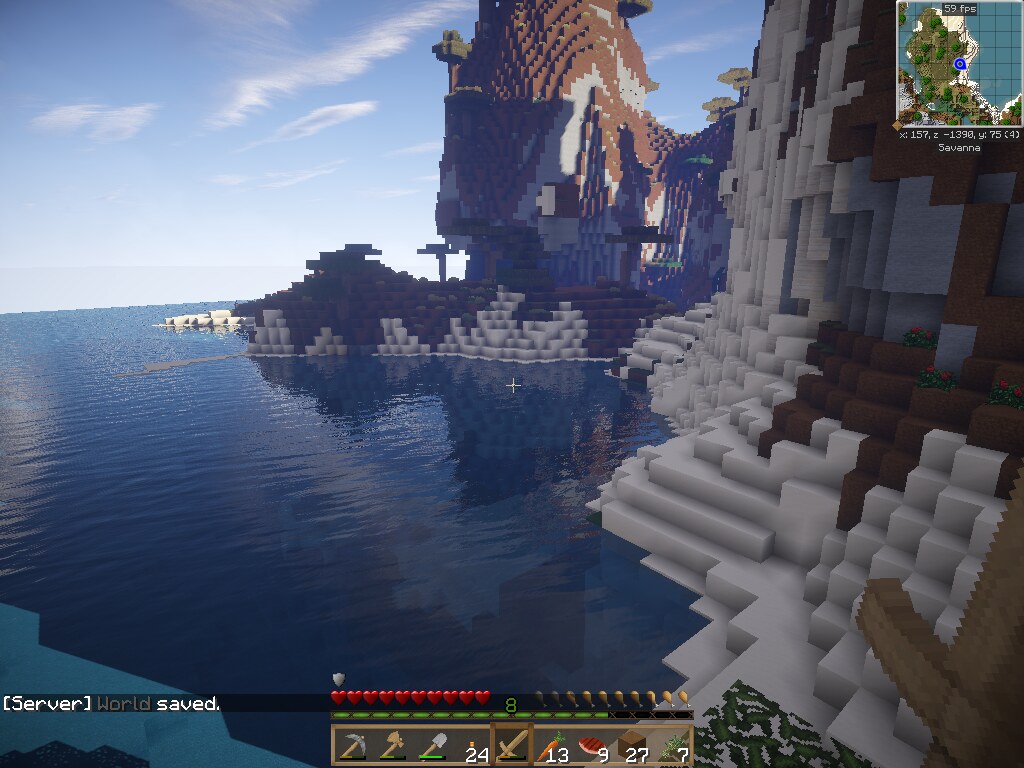The image showcases a digital game interface with significant similarities to Minecraft. The primary scene features an expansive ocean on the left side, transitioning into a landscape of blocky mountains and potential structures, typical of voxel-based environments. The game's heads-up display (HUD) at the bottom of the screen displays various player statistics, including food and health levels. Icons indicating the player's inventory, such as swords, shovels, and other tools, are also visible. A message at the bottom reads "Server world saved," indicating a recent save point. In the top right-hand corner, a mini-map marks the player's current location by the ocean, amidst dirt terrain.